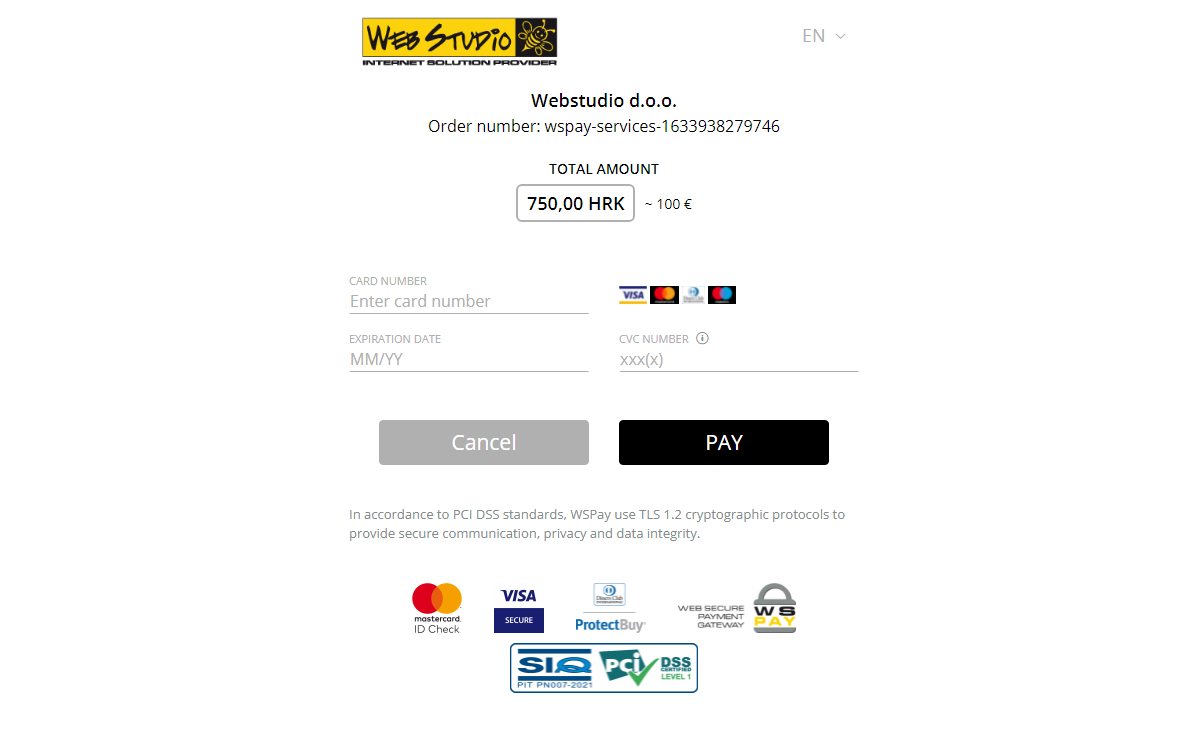**Web Studio - Internet BOLUtion Provider Interface**

The top of the interface features a banner with the text "Web Studio" in bold, set against a yellow background. Nearby, there's an outlined drawing of a honey bee in yellow, symbolizing productivity and connectivity. Directly above, you'll find the title "Internet BOLUtion Provider."

On the right side, there is a language selector denoted by "EN" in gray, accompanied by a drop-down menu for changing the language settings.

Beneath the banner, the text "Web Studio Order Number" is displayed, followed by a specific identifier: "WSPAYDASS1633938279746". This likely serves as a unique order identifier.

Further information about the transaction includes:
- **Total Amount**: 750,000 HRK (displayed prominently)
- Following this is convoluted text suggesting a conversion or an additional amount, resembling "Dash 100," possibly hinting at a value in euros (€100).

For payment details, the form requests:
1. **Card Number**: Instruction to "enter card number."
2. Options for entering card details include logos for Visa, MasterCard (appearing twice), and Diners Club.

Additional fields to be completed are:
- **Expiration Date**: Separate fields for month and year.
- **CVC Number**: Request to provide the card verification code, masked for security.

Two buttons conclude the form interface:
- **Cancel** (colored gray)
- **Pay** (colored black)

Below these buttons, there’s a note ensuring compliance with industry standards:
"In accordance with PCI DSS standards, WSPAY uses TLS 1.2 cryptographic protocols to ensure secure communication, privacy, and data integration."

Finally, security features and certification icons are lined up at the bottom:
- **MasterCard ID Check**
- **Visa Secure**
- "Protected by Web Service Payment Gateway WSPAY" affirmation
- Authentication and certification numbers: “PNSQIPTPN00072021” and “DSS Certified Level 1 PCI”.

This detailed description lays out the specifics of the payment interface provided by Web Studio, ensuring users about the secure and standard-compliant environment they've established for processing transactions.